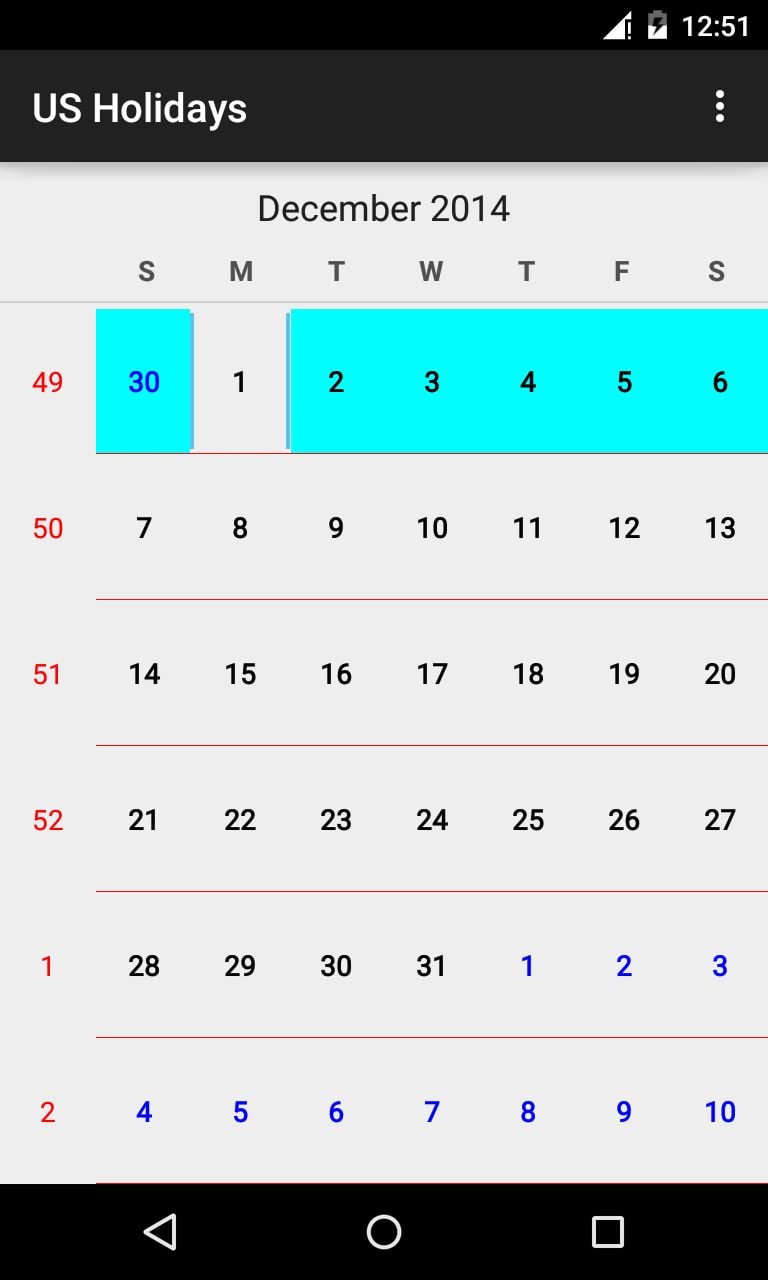In this image, an Android phone screen displays a retro-styled calendar app set to December 2014. The calendar features a plain grey background and highlights each week of the year, with the final week labeled "52." Notably, the dates from November 30th and December 2nd through December 6th are highlighted with an aqua-colored background, suggesting these dates have events marked. Regular calendar digits appear in black, while upcoming dates in January are shaded in blue. The calendar follows a Sunday through Saturday weekly format, looping back at week's end. Additionally, the phone's status bar indicates a cell signal that appears to be non-functional and a battery level at approximately 50%.